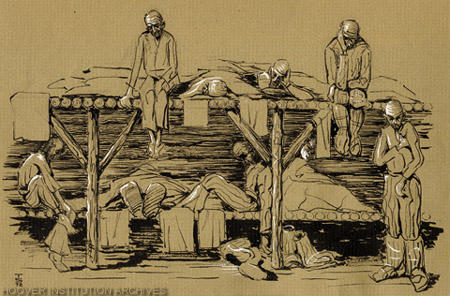This image is an illustration, possibly a drawing or a print, showing a brownish-tan scene detailed in black or dark brown. The focal point is a primitive wooden structure, resembling bunk beds or a log loft, supported by vertical poles. There are six to eight people positioned on these structures and logs. Three individuals are on the upper portion, with two sitting at the edge and one standing at the right, facing forward. On the lower bunk, there are two more individuals, and possibly another person beneath, partly obscured. All the individuals appear to be fully dressed, reclined, or sitting in various positions, projecting a sense of fatigue or melancholy. Their expressions and postures indicate sleepiness, sadness, or illness. Two logs are visible at the front center, contributing to the overall rustic appearance of the scene. Text at the bottom left reads "Hoover Institution Archives."